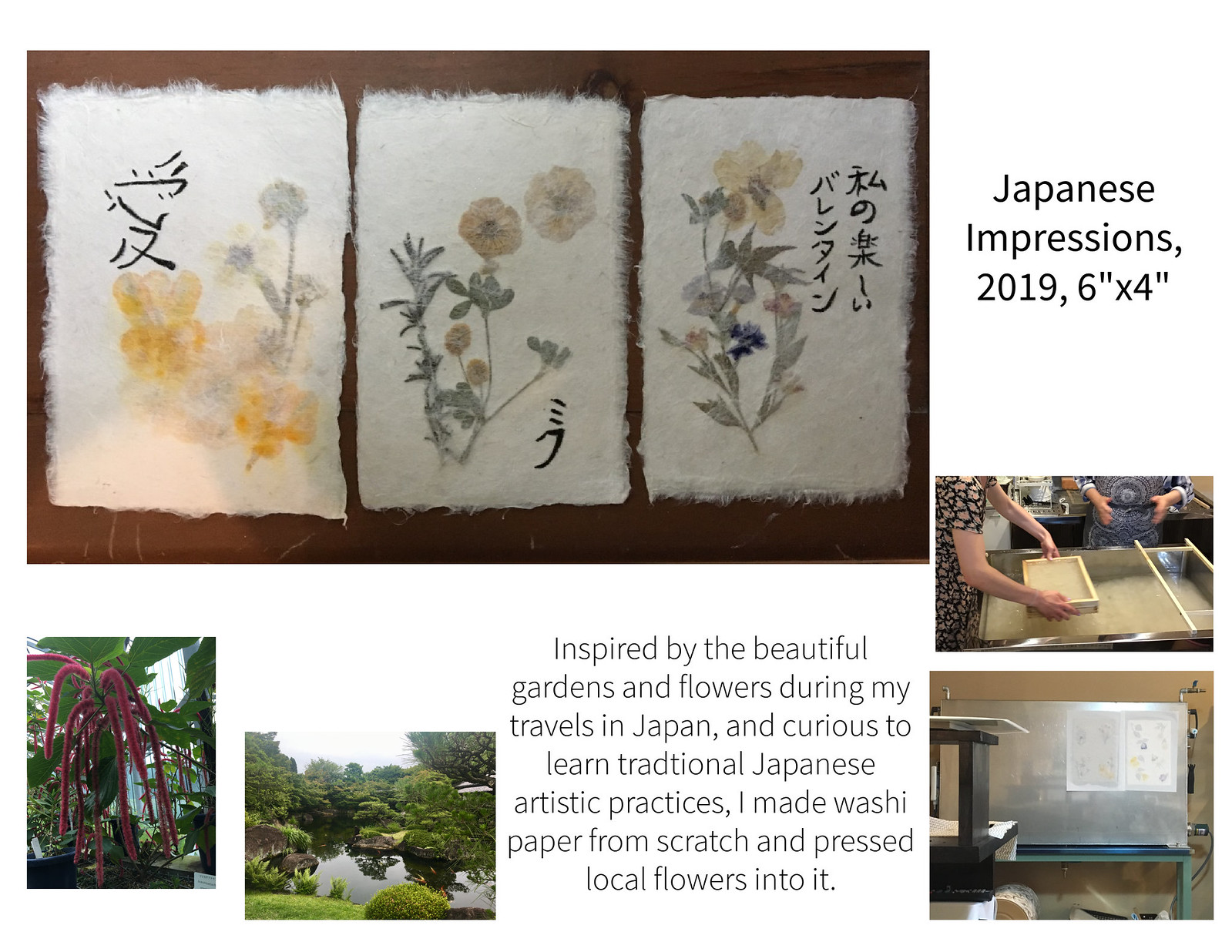The central image, titled "Japanese Impressions 2019, 6x4," showcases three Japanese Impressionist pieces created on washi paper, featuring impressions of actual flowers left behind on the paper, instead of painted representations. This collection was inspired by the beautiful gardens and flora observed during travels in Japan and created through a traditional Japanese artistic practice of making washi paper from scratch and pressing local flowers into it. Below this central image, accompanying text explains the process and inspiration. In addition, the bottom-left section contains two photographs displaying local Japanese vegetation: one capturing a vibrant red flower and another depicting a marshy garden landscape. On the right, two more images illustrate the traditional paper-making process: one showing wooden frames about to be submerged in a vat, and another displaying sheets of washi paper hanging to dry. The entire description is presented in a clean, black font.